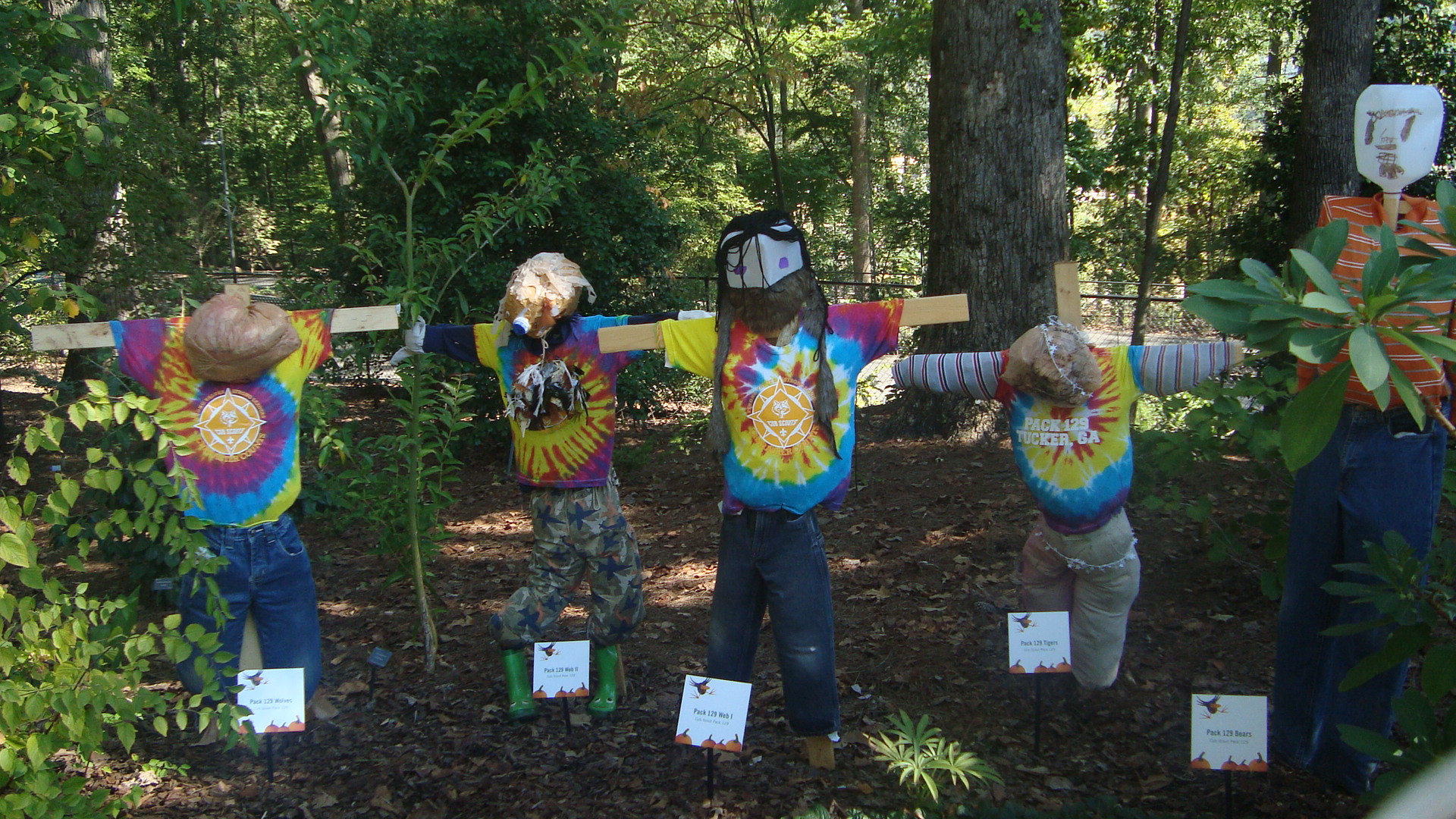In a vibrant garden enclosed by a black gate, a unique array of scarecrows stands guard. The garden is adorned with small green leaves on the left side and longer, wider leaves on the right, with thick-trunked trees providing a lush backdrop. The ground is a mix of brown grass, dirt, and scattered dead leaves. Central to the scene, several scarecrows made of wooden crosses and legs are dressed in brightly colored tie-dye shirts, with one exception in an orange and white striped shirt. From left to right, the shirts display vivid hues of yellow, purple, blue, and red, each adorned with various logos. One notable tie-dye shirt on the far right reads "PAC-429 Tucker GA," paired with a long-sleeve striped shirt underneath, while another scarecrow sports blue jeans. Among the scarecrows, there are both child-sized and adult-sized figures, with paper faces drawn on two of them, and others topped with hats. A gray chain-link fence is visible at the horizon, demarcating the end of the garden and the beginning of the wooded area gracing the background.